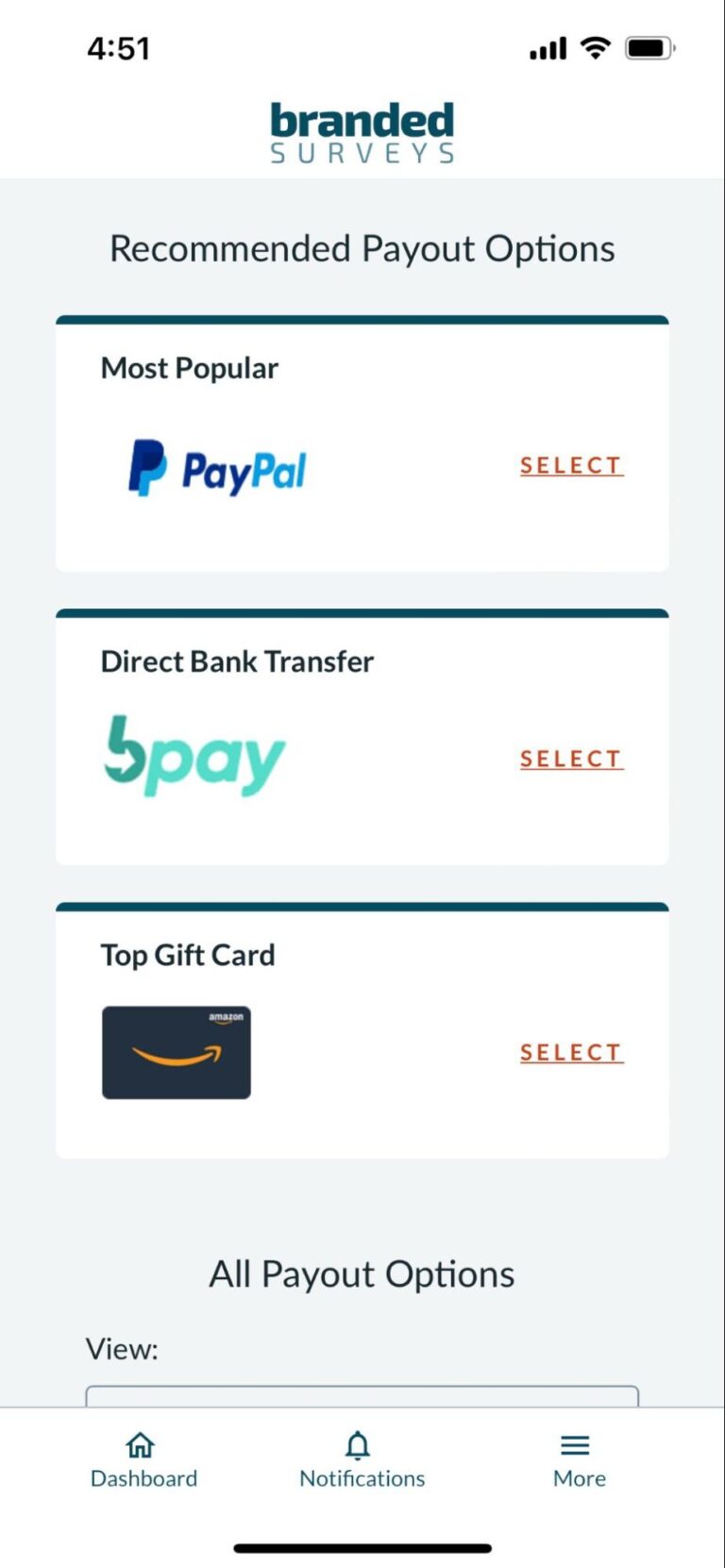The screenshot depicts a smartphone screen showcasing a webpage from "Branded Surveys." The user appears to be on the "Recommended Payout Options" section, likely indicating that they have accumulated earnings from completing surveys and are now exploring ways to cash out. The page prominently displays three most popular payout methods:

1. **PayPal:** Accompanied by its recognizable logo and a red 'Select' button.
2. **Direct Bank Transfer:** Indicated by the BPAY logo, also with a red 'Select' button.
3. **Top Gift Card:** Featuring an Amazon gift card image and a red 'Select' button.

Below these options, there is a partially visible section labeled "All Payout Options," suggesting additional methods are available but require scrolling to view.

At the top of the screen, standard smartphone icons are displayed, showing the time, signal strength, and battery level. The app's navigation bar at the bottom includes three menu items: "Dashboard," "Notifications," and "More."